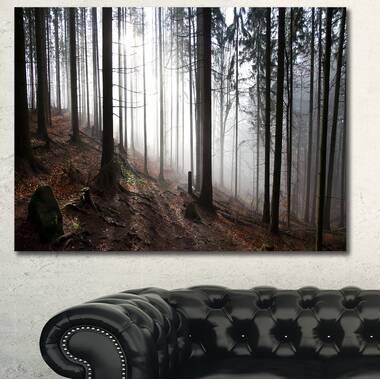The image depicts a cozy family or living room with a photograph or painting mounted on a gray, cement-like wall. The artwork, which is rectangular and prominently displayed above a low-backed black leather couch with beaded, bubble-like detailing, captures a forest scene on a foggy, steep hillside. The hillside slopes from the taller lower left corner to the lower right. Tall, partially bare trees, likely pine trees, are scattered amid large rocks. A dense fog or mist permeates the forest, creating a white halo glow that suggests the sun is rising, casting a muted light through the trees and producing elongated shadows. The overall ambiance is serene and captivating, drawing attention to the contrast between the dark, intricate details of the trees and the ethereal brightness of the misty background.